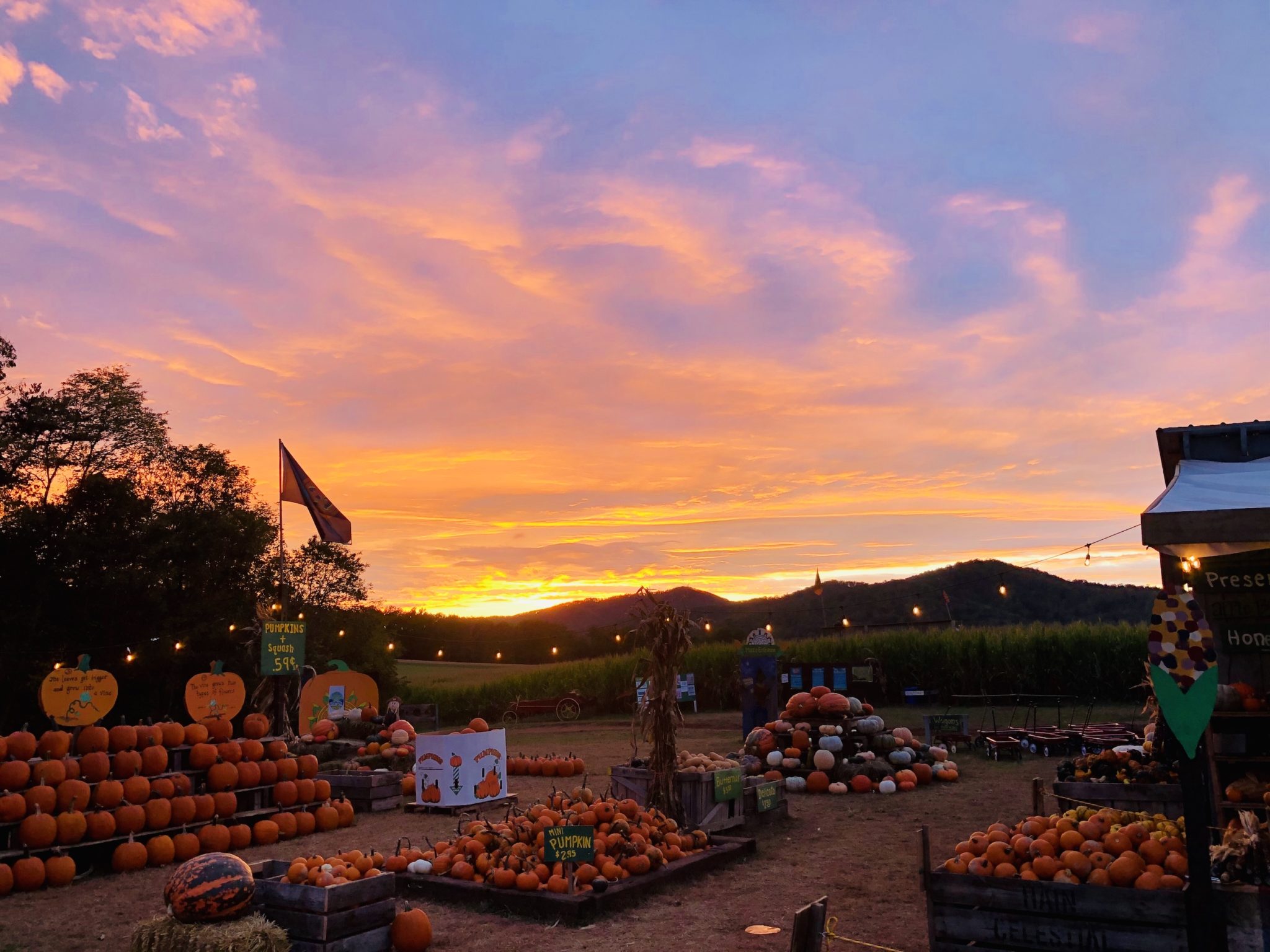In this captivating photograph of a pumpkin patch taken during a beautiful sunset, vibrant oranges and warm hues bathe the scene, creating a picturesque ambiance. The patch is set in a courtyard surrounded by trees and tall grass, with a breathtaking sky transitioning from blues to oranges and yellows as the sun dips below the horizon. There's an organized display of pumpkins, most of which are orange, with some uniquely colored in gray, black, yellow, and even red and green. 

In the foreground to the bottom left, an orderly shelf or rack, arranged like bleachers, holds several pumpkins, while to the right, smaller pumpkins are gathered in a large wooden basket. Out in the open, a massive pile of pumpkins of all shapes and sizes draws attention, alongside some standalone giants. Overhead, a string of twinkling lights adds to the festive atmosphere, and various flags, including a prominent red one, flutter gently in the evening breeze.

Scattered throughout the patch are little vending stalls, featuring piles of tiny pumpkins and other produce, like tomatoes. An intriguing sign reading "squid 59 cents" and pumpkins adorned with drawings and writings are also visible, although the specifics of the writings remain unclear. The entire scene is suffused with a brownish-gold light from the setting sun, enhancing the magic of this autumnal tableau.